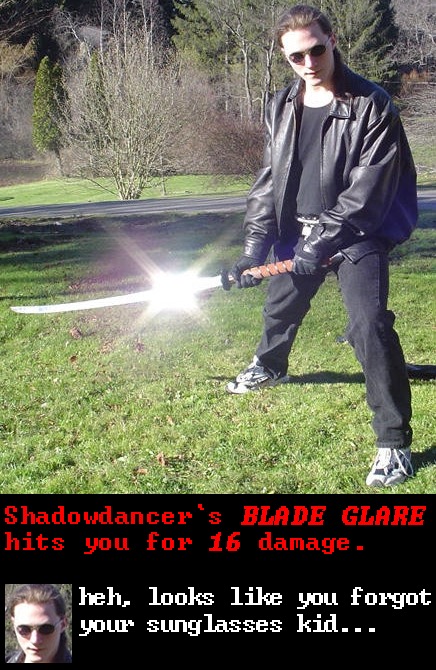The image is a meme photograph depicting a light-skinned man standing in a grassy park area under a sunny sky. The man, who has brown hair pulled back to his shoulders, is dressed in a black leather jacket over a black shirt, black jeans, and black-and-white shoes. He is wearing black gloves and sunglasses, which add to his somewhat formidable appearance. He is holding a large katana with a brown hilt in both hands, and the blade, which shines brightly in the sunlight, extends from the center of the image to the left, creating a noticeable glare. Behind him, there is a pathway, likely made of concrete or asphalt, and several trees with a mix of green leaves and bare branches fill the background. The meme text at the bottom of the image reads in red, "Shadow Dancer's Blade Glare hits you for 16 damage," with a smaller caption in white below, "Hey, looks like you forgot your sunglasses, kid." To the bottom left, there is a cut-out of the man's face echoing the same phrase, emphasizing the humorous, game-like nature of the meme.